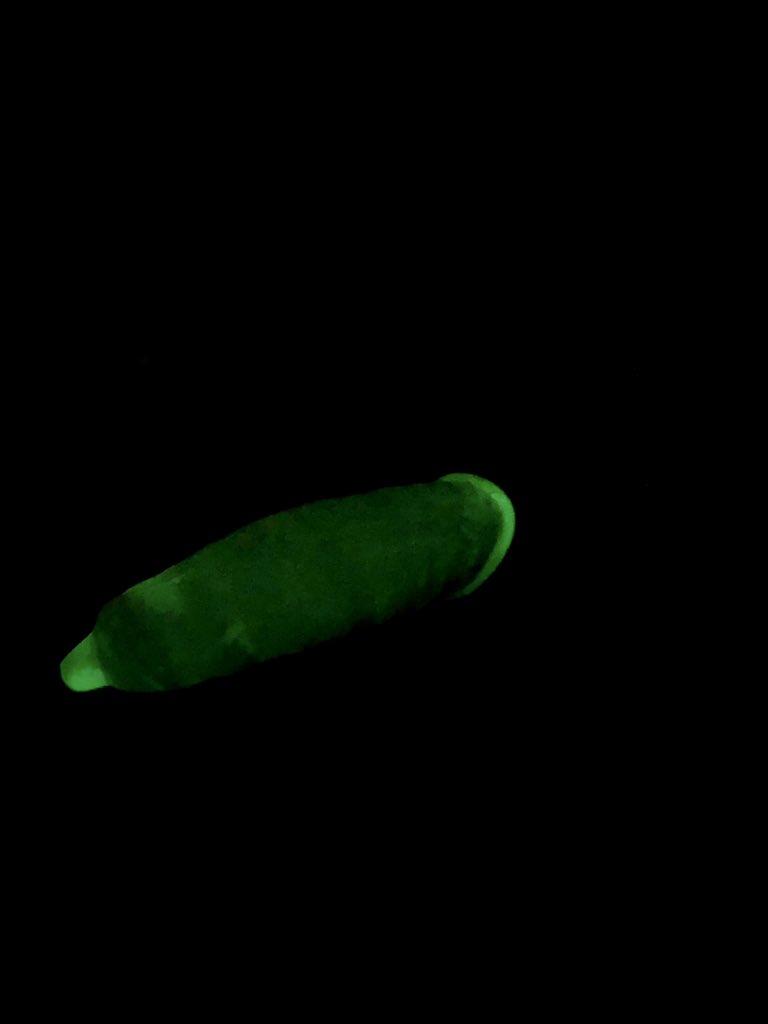The image is a vertically rectangular photograph with no border, featuring a solid black background. In the center, there's a small, dark green, tube-shaped object resembling a caterpillar or a cucumber, oriented slightly diagonally from bottom-left to top-right. The object is notable for its bioluminescent qualities, with both ends glowing a vivid neon green. The left end is narrower, almost shaped like a nipple or a gumdrop, while the right end is wider with a backward C-shaped highlight. The rest of the object shows lighter green patches, giving an impression of translucency, as if light is filtering through its skin. The glowing ends give the impression of an animal with bioluminescent features, possibly a deep-sea creature.